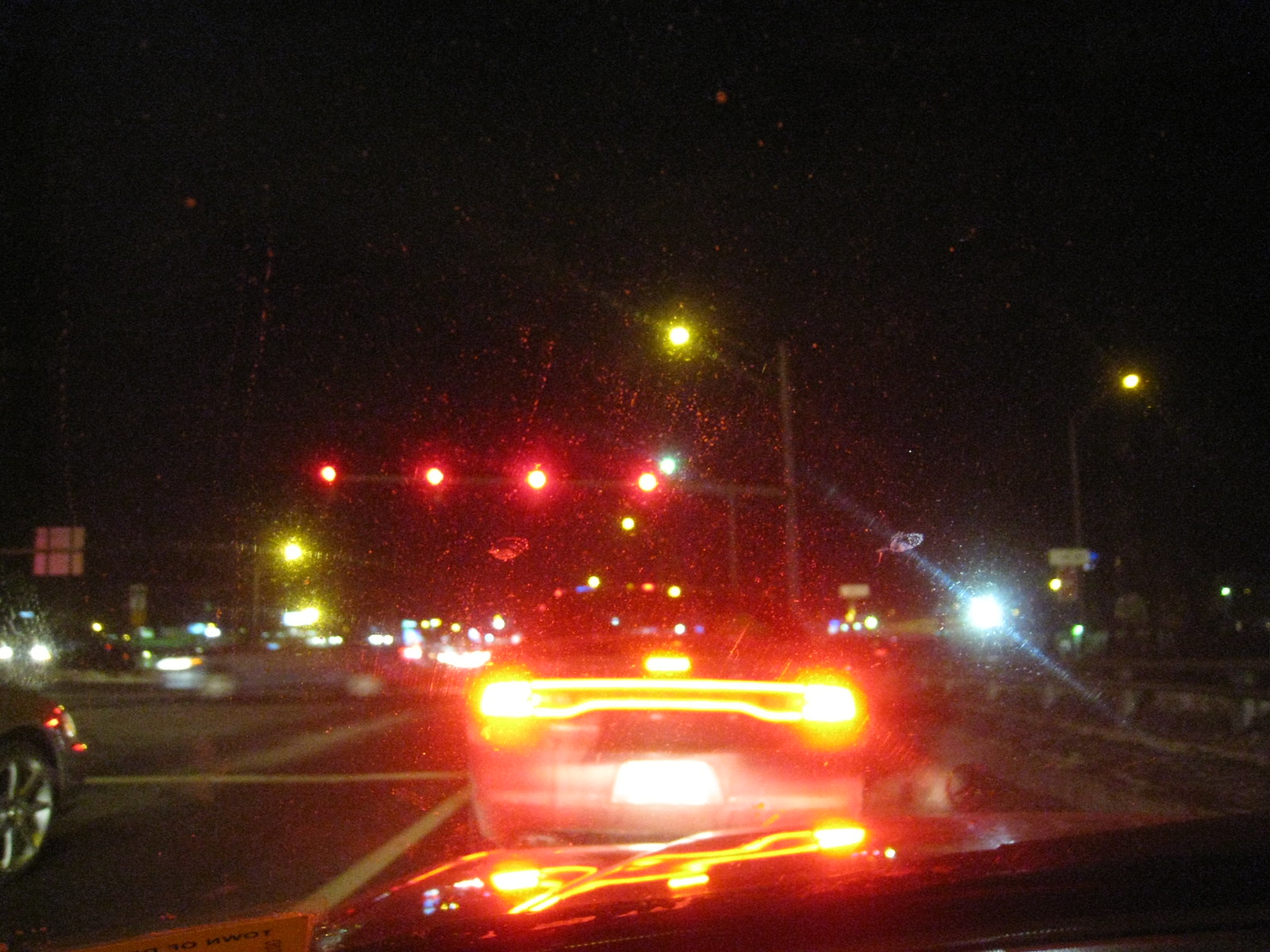The image captures a scene of a bustling urban intersection on a very dark night, as viewed from the perspective of a driver inside a car. The windshield frames the scene, revealing a few streetlights casting a yellow glow on the busy road ahead. Directly in front of the car is another vehicle, its brake lights shining brightly. To the left, a car has just emerged from a side street, turning left and crossing the driver's path. A prominent pole with a horizontal arm holds four traffic lights, all illuminated in red. Off to the right, a glare reflects off what appears to be a glass door of a building, hinting at the surrounding commercial district. The scene is dense with urban ambiance, characterized by its nighttime cityscape and active traffic.